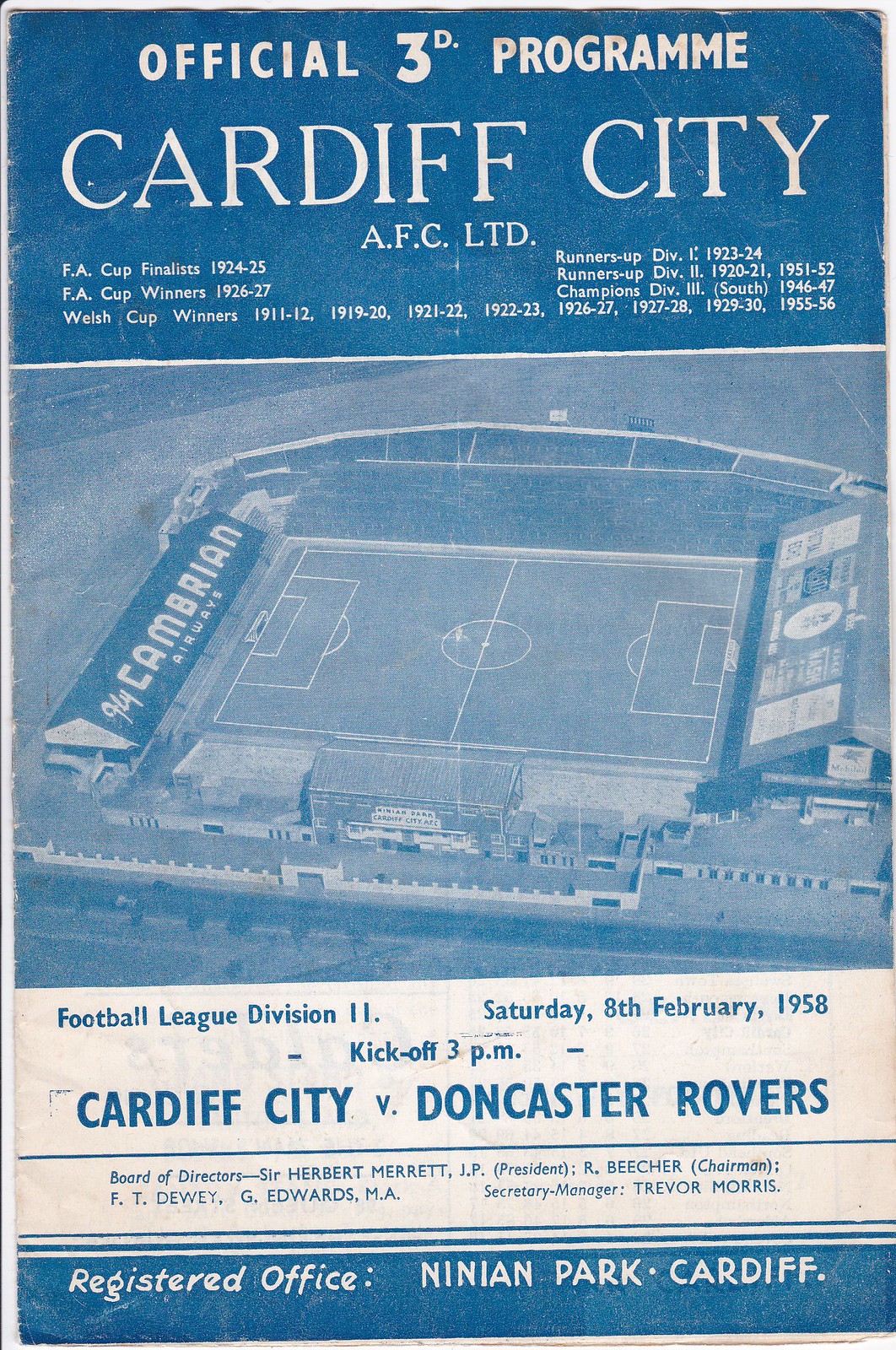The cover of the program for the Cardiff City Soccer Club, set against a predominantly medium blue background, prominently features the title "Official 3rd Program" in white at the top. Beneath this, in smaller white text, it reads "Cardiff City AFC Ltd," followed by a list of their notable achievements, including being FA Cup finalists and runners-up, with a special note on them winning the FA Cup in 1926-27. 

Centrally, there's an aerial photograph of the stadium, with gray grass marked by white lines and surrounded by spectator stands, a scoreboard, and an advertisement displayed at one end of the pitch. 

The bottom section shifts to a white background with blue lettering detailing the match information: "Football League Division II, Saturday, 8th February, 1958, Kickoff, 3 p.m. - Cardiff City v. Doncaster Rovers." The very bottom of the cover features a blue border with white text stating "Registered Office, Ninian Park, Cardiff."